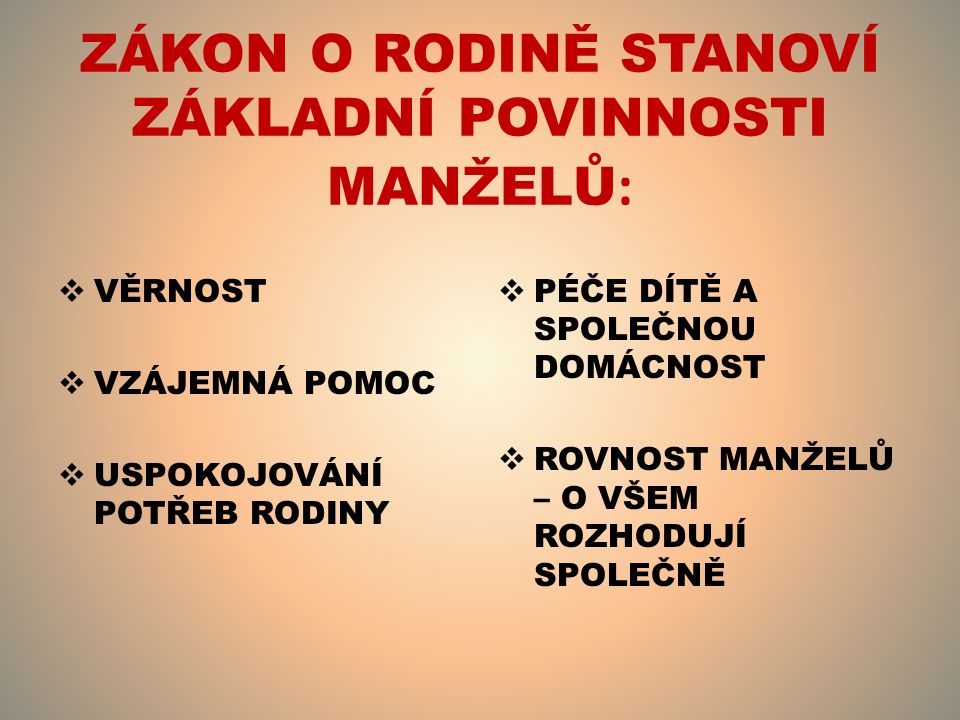The image appears to be a slide from a PowerPoint presentation, written in an Eastern European language, possibly Hungarian or Polish. The title text is prominently displayed at the top, centered and in bold red uppercase letters: "ZAKON O RODIN STENOVI." Below the title, the slide contains additional text in black uppercase lettering, organized into five bullet points. Three of these bullet points are aligned in a column on the left side, while the remaining two are positioned in a column on the right. The background is predominantly brown, transitioning to a brighter golden hue towards the center, giving the impression of sunlight shining from behind. The slide is neatly formatted with a focus on text, and does not include any images or other objects.